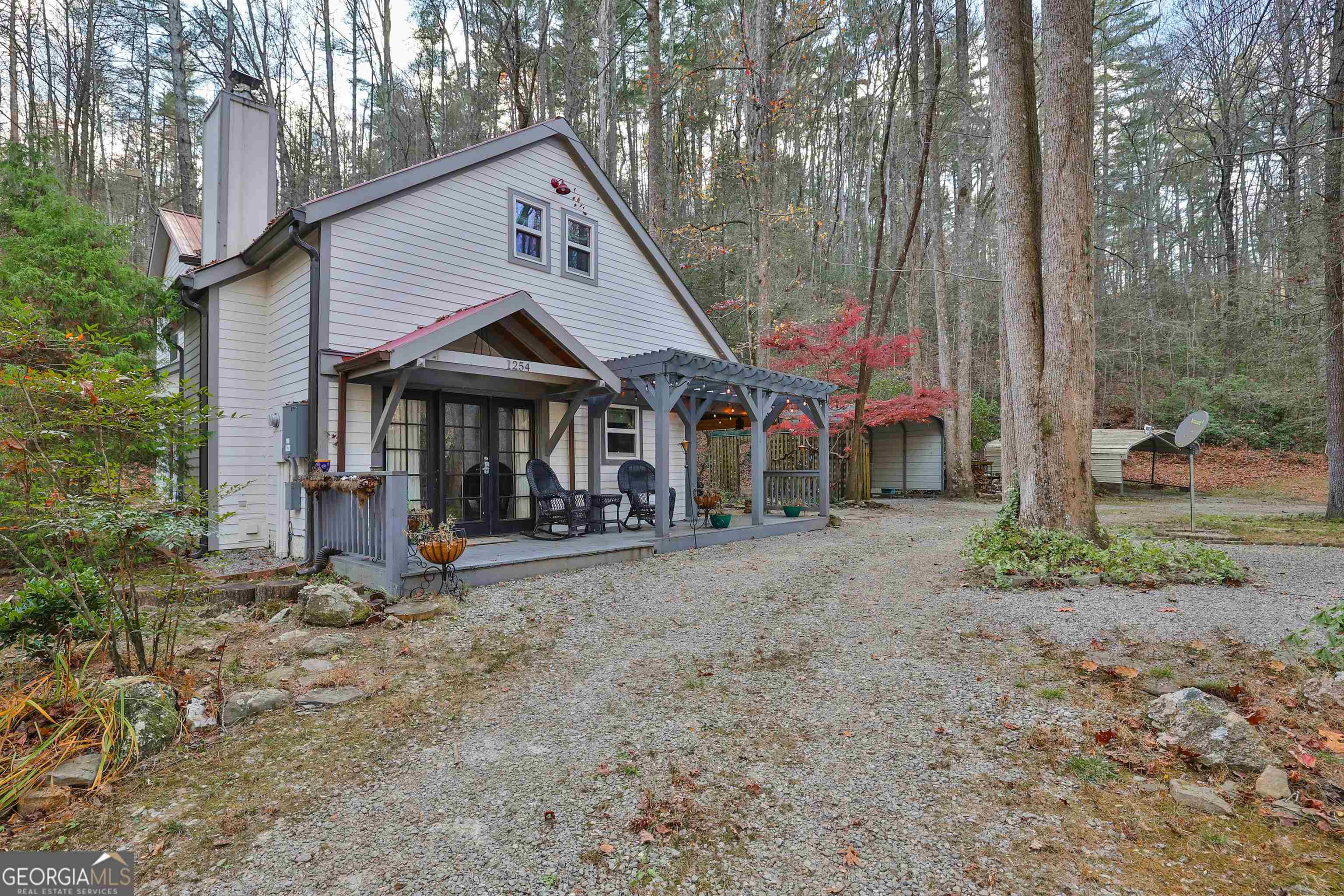This photograph depicts a quaint house set in a rustic, wooded landscape. The house features light gray siding with darker gray trim and a striking red, possibly metallic, roof. Its structure includes multiple roof points, a plain chimney on the left side, and a steeply sloped roof with a central red hanging lamp between two front windows. The front porch, painted dark grayish blue, hosts two black wicker rocking chairs and two green plant pots, alongside two baskets filled with an orange substance. A gravel pathway, marked by a brown stripe, leads up from the bottom of the frame to the house, flanked by rocks and green plants on the left and gray rocks on the right. Prominent on the right is a large light brown tree trunk with green leaves underneath. Distant pale, barren trees suggest it's fall, echoed by a bright red tree near the two slightly arched metal sheds to the right of the house. A satellite dish is visible at the far right, rising from the gravel driveway.